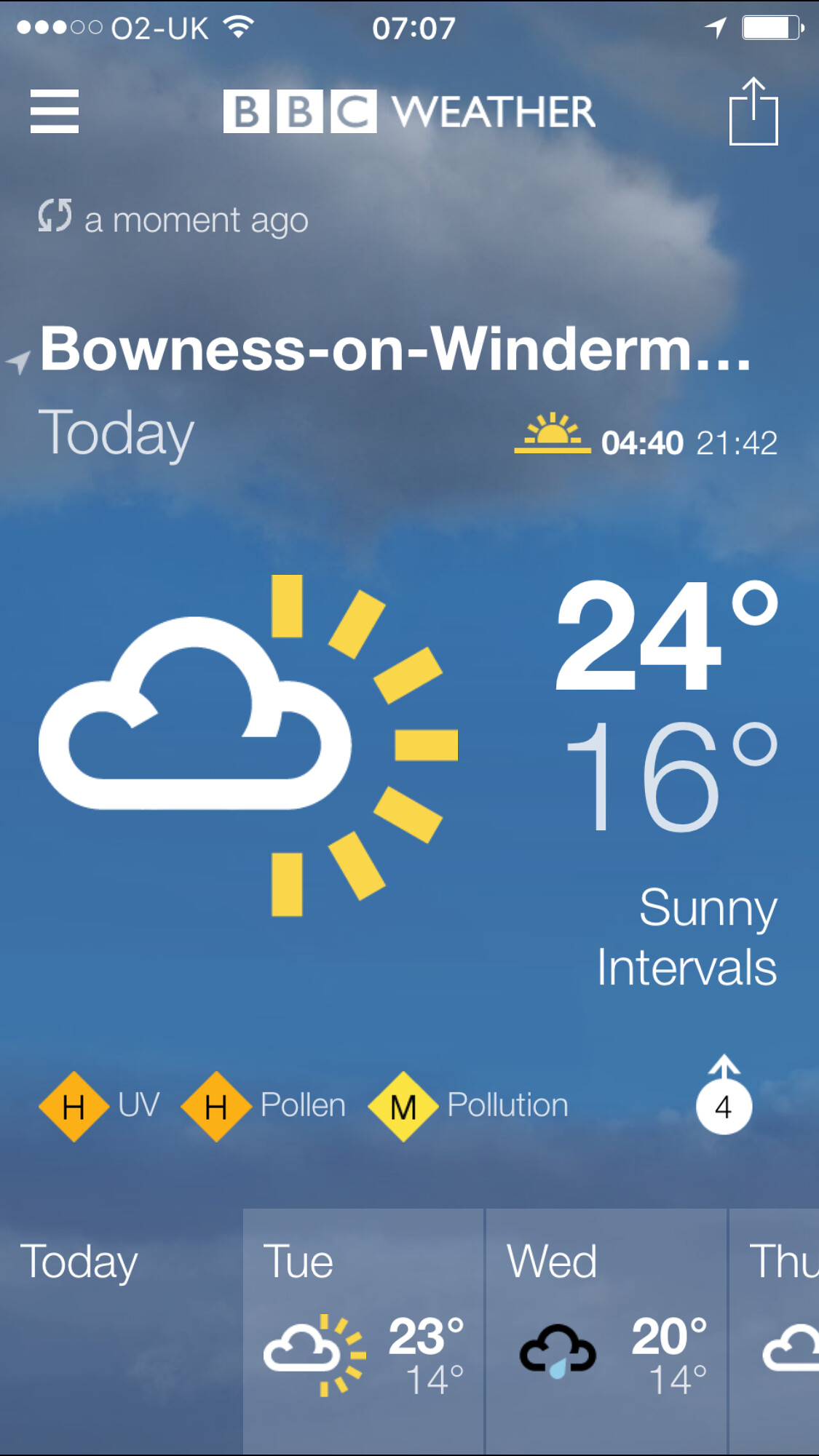This detailed color screenshot from the BBC Weather app captures various weather details for Bowness on Windermere, although part of the town name is cut off. At the top, the BBC Weather logo is prominently displayed, alongside information indicating a recent refresh and typical phone status icons — Wi-Fi signal, time, and a partially drained battery. For the current day, it shows the time at 4:40 PM with a temperature reading of 24°C (16°C for the low), depicted with a sunny intervals icon featuring a cloud with sunbursts. Below, it provides alerts for high UV levels, high pollen count, and medium pollution levels, symbolized by three diamonds. The extended forecast includes weather predictions with symbols: Tuesday’s forecast indicates partly cloudy with a high of 23°C and a low of 14°C, Wednesday predicts rain with similar temperatures, and Thursday's information is partially cut off but suggests cloudy weather.